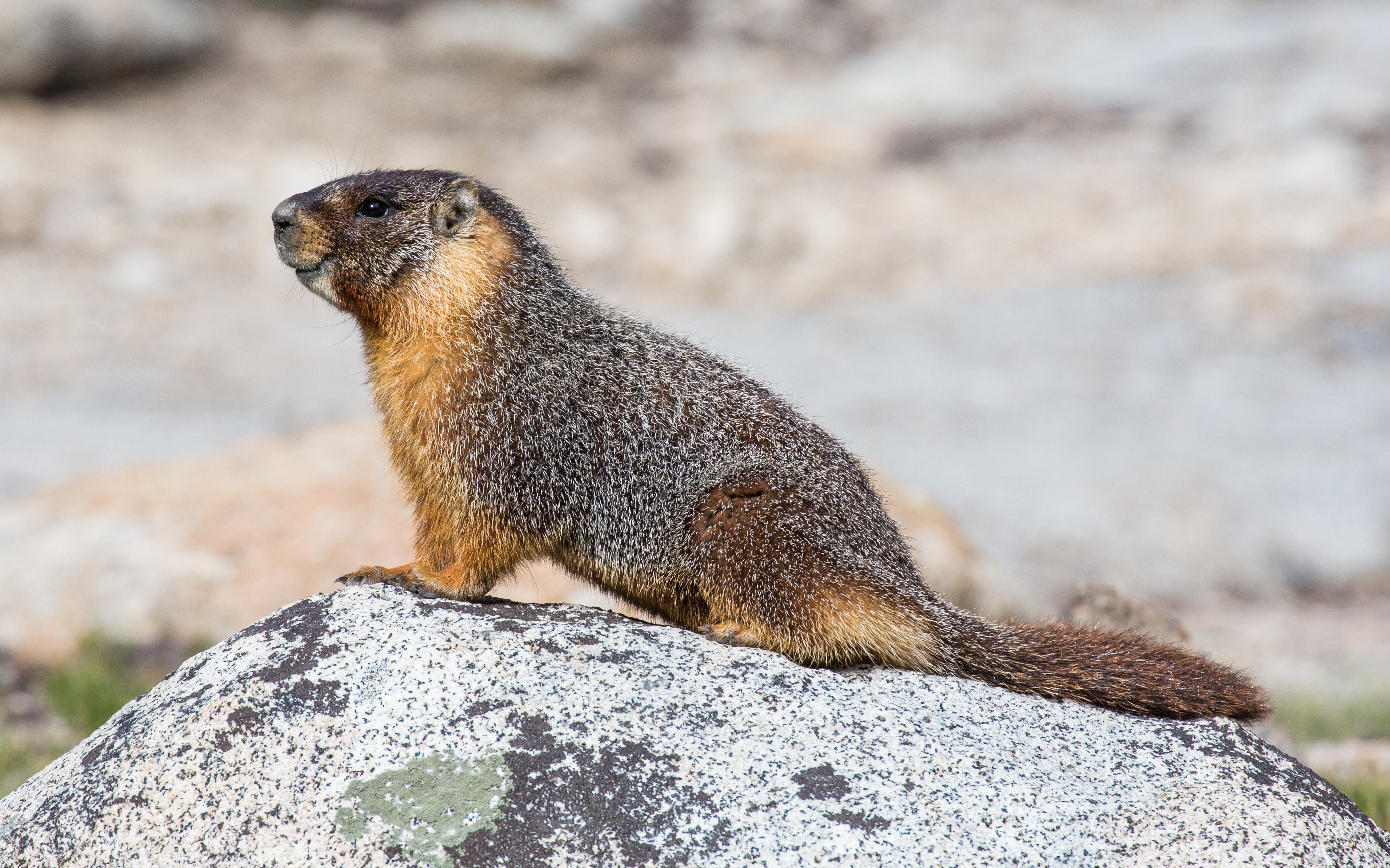A small, inquisitive mammal, potentially a young beaver, is perched on a well-worn rock, sitting on its haunches with its forelegs upright. The creature gazes ahead, its expression almost resembling a smile. Its fur is predominantly gray, interspersed with salt-and-pepper shading that gives it a snow-dusted appearance, although there's no actual snow present. Its chest and forelegs are a contrasting tan color. The creature's flat tail is partially visible, contributing to the identification as a possible beaver. The rock on which it sits is eroded, likely by the wind, and features a small, green patch that could either be lichen or part of the rock's natural coloring. Surrounding this contemplative mammal is a stark, rocky landscape with minimal vegetation, suggesting a sparse, yet captivating environment. Despite the barren scene, the proximity of water is implied by the animal's presence. The detailed textures and colors in both the mammal's fur and the geological features create a serene and intriguing snapshot of nature.